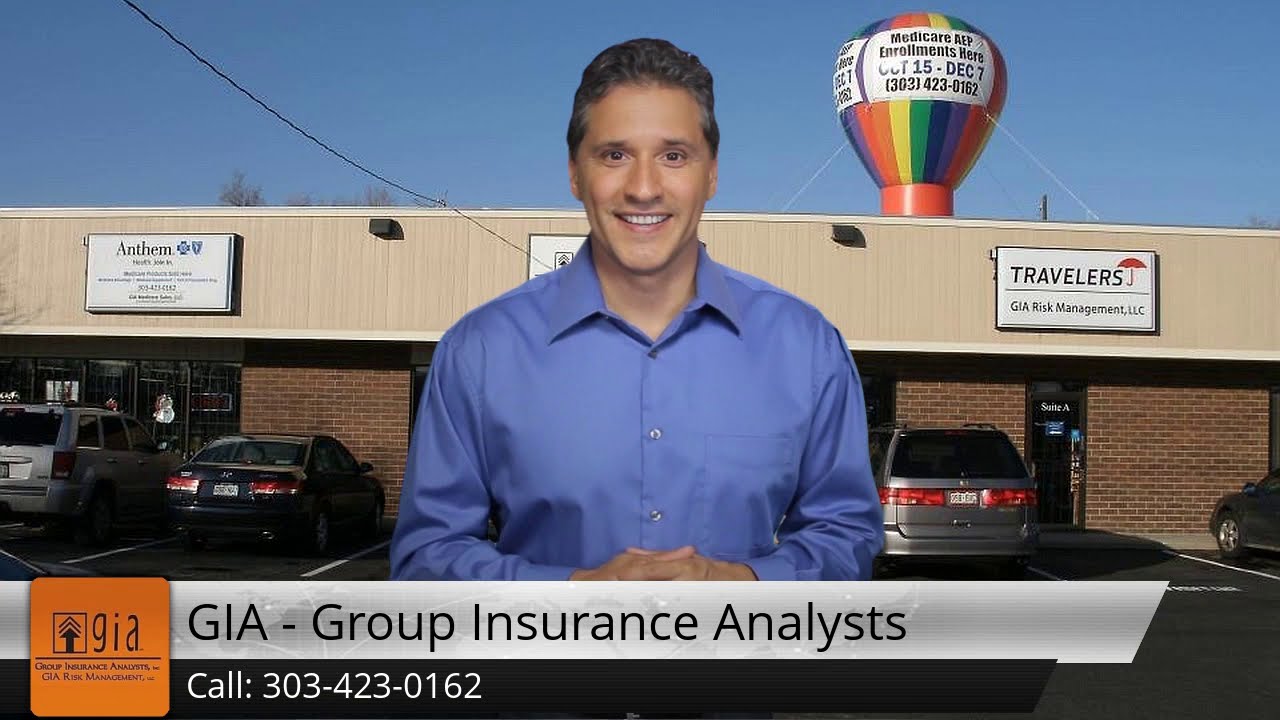In the image, a man stands front and center in a strip mall parking lot, smiling warmly at the camera. He is a middle-aged white man dressed in a light blue button-up shirt. The man appears superimposed onto the background, suggesting a graphical element. Behind him, the strip mall houses several businesses, including Blue Cross Blue Shield Anthem and Travelers Insurance. Parked vehicles are visible in front of the buildings. Dominating the background is a large, rainbow-colored hot air balloon with text advertising Medicare enrollment dates from October 15th to December 7th. At the bottom of the image, a rectangular banner reads "GIA - Group Insurance Analysts," featuring their logo—a yellowish square—and a contact phone number, 303-423-0162. The sky above is clear and blue, adding a sense of openness to the busy and detailed scene.